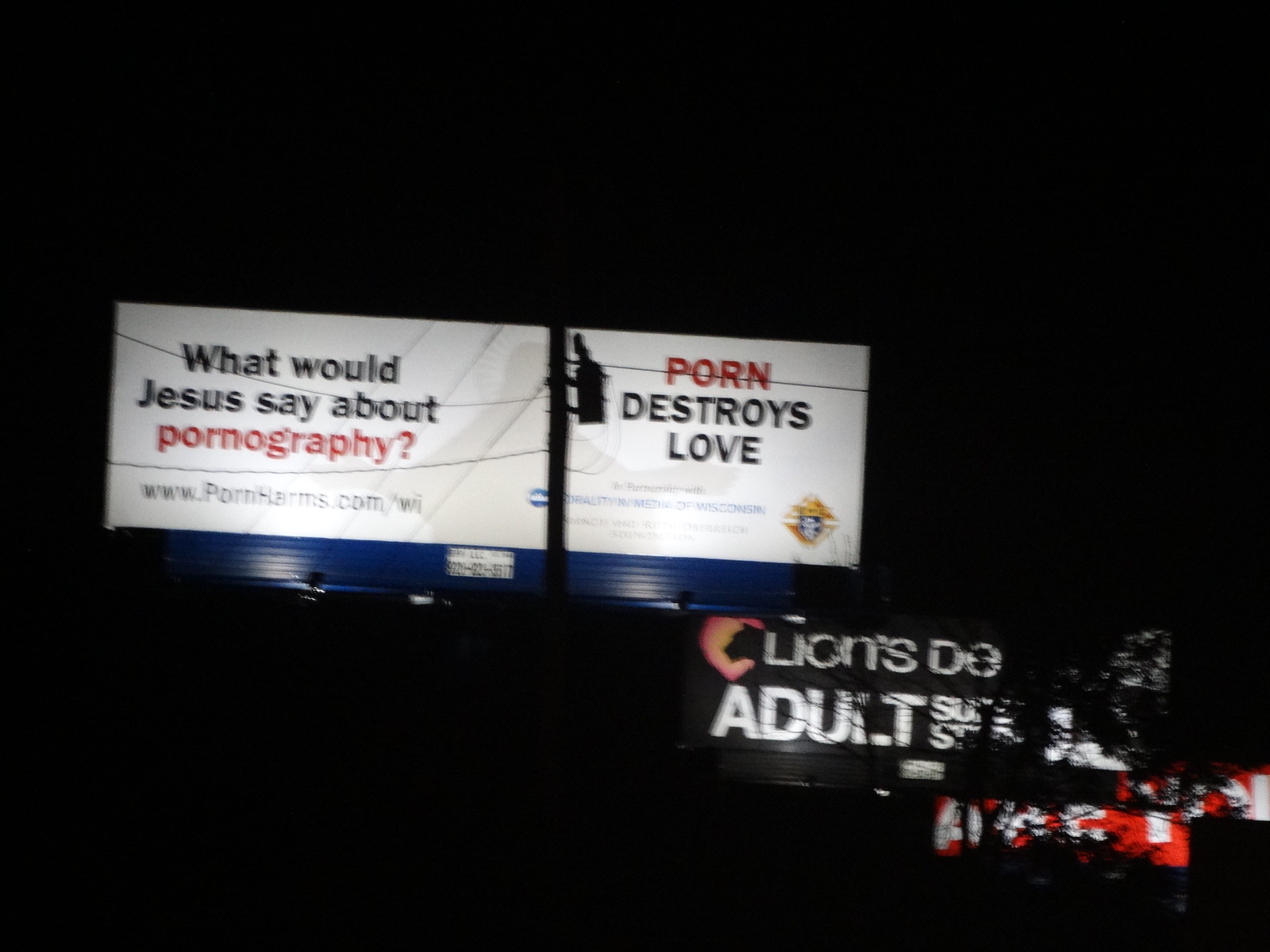This nighttime color photograph centers on a stark white billboard displaying a provocative message: "What Would Jesus Say About Pornography? Porn Destroys Love, www.pornharms.com/W-I." This thought-provoking text occupies the middle section of the billboard. Below this, another billboard advertises the Lion's Den Adult Superstore, contrasting sharply with the anti-pornography message above. To the bottom right of the image, a hint of red taillights is visible, implying nearby traffic. The sky is pitch-black, providing a dramatic and intense backdrop. Notably absent from the scene are people, animals, buildings, and any form of vegetation, leaving the billboards as the sole focal points in an otherwise empty landscape.